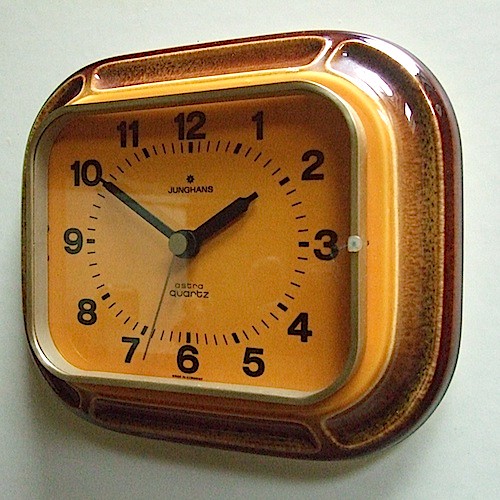The image depicts a clock mounted on a white wall. The clock has a striking design, featuring a square shape with rounded edges and appears to be constructed of a ceramic or pottery-like material with a high-polished, dark brown speckled finish. The clock face itself is orange with bold black numbering and three black hands for the hours, minutes, and seconds. The exact time displayed is 1:50, with the seconds hand slightly past the 34 second mark. Notable inscriptions on the clock face include "Junghans" and "Astra Quartz," indicating the brand and type. Overall, the clock exudes a blend of vintage charm and modern craftsmanship.